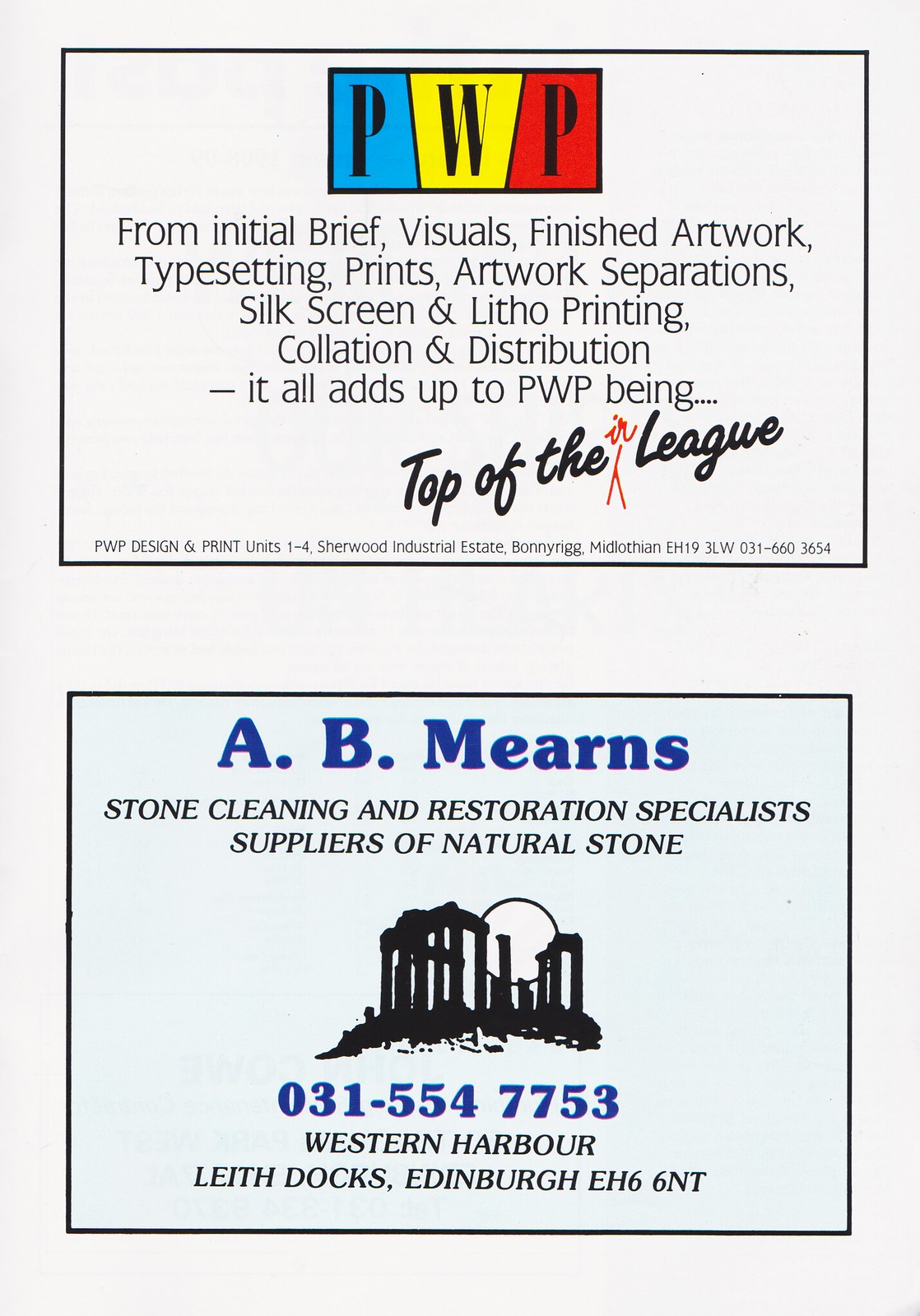This page, reminiscent of a magazine or newspaper layout, features two black rectangle-box advertisements on an off-white background. The upper advertisement showcases a vibrant combination of blue, yellow, and red rectangles with the letters "PWP." Below in black typography, it details the services: from initial brief and visuals to finished artwork, typesetting, artwork separation, silkscreen, and litho printing, along with collation and distribution. The caption emphasizes that all these components contribute to PWP being at the top of the IR League, and includes their address and phone number: PWP Design and Print, Units 1-4 Sherwood Industrial Estate, Bonnie Rigg, Middleton EH19 3LW, 031-6603654.

The lower advertisement highlights A.B. Mearns, a specialist in stone cleaning and restoration, and a supplier of natural stone, depicted through an illustration featuring a classical marble column scene against an ancient Grecian backdrop with a moon. Contact details are provided: A.B. Mearns, Western Harbour, Lee Docks, Edinburgh, EH6 6NT, 031-554-7753.